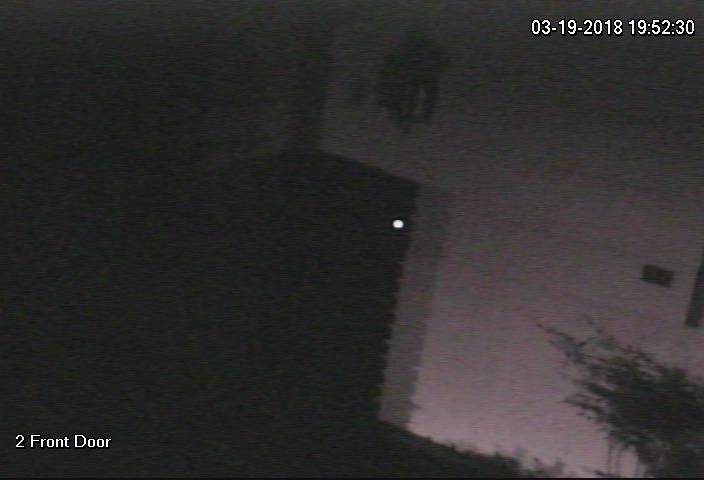The image, taken from a security camera at nighttime, captures an outdoor scene dominated by dark shades and minimal lighting. At the top center, white text displays the date "03-19-2018" and the time "19:52:30". The left side of the image is shrouded in darkness, making it difficult to identify specific details. Moving towards the center, the scene becomes slightly more illuminated, revealing possible white walls and the silhouette of a door or a garage door with an indistinct object hanging on it. On the right side, the silhouette of a tree with long branches or leaves is visible, partially casting shadows on the wall. At the bottom right corner, more text, reading "2 FRONT DOOR", is printed in white. The background sky transitions from a gray to a lighter gray-purple hue, enhancing the eerie ambiance of the nighttime image.